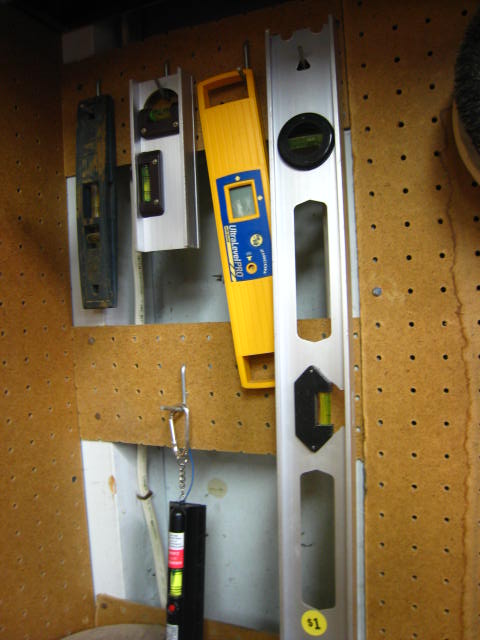In the image, there is a section of what appears to be a hardware store or a personal workshop area dedicated to hardware and machinery. The background features a brown, cardboard-like surface with numerous small nail holes, suggesting frequent use or a makeshift display.

On the top rail, four distinct items are neatly arranged:

1. The first item is a dusty, blue rectangular device, the specific function of which is indeterminate due to the dust obscuring details.
2. The second item is a small, silver rectangular object featuring a circular opening at the top. A black piece is attached to its top, adding to its complexity.
3. The third item is a vibrant yellow, elongated rectangle with a central blue section that houses a small screen, bordered in yellow.
4. The fourth item resembles an elongated version of the second item. It is primarily silver with black components, including a small screen and several openings, one in the center and another at the bottom.

On the bottom rail, there is a black item adorned with a chain and a hint of color, adding a functional and possibly decorative touch to the setup. Overall, the image captures a mix of tools and machinery, meticulously organized yet indicative of active use.